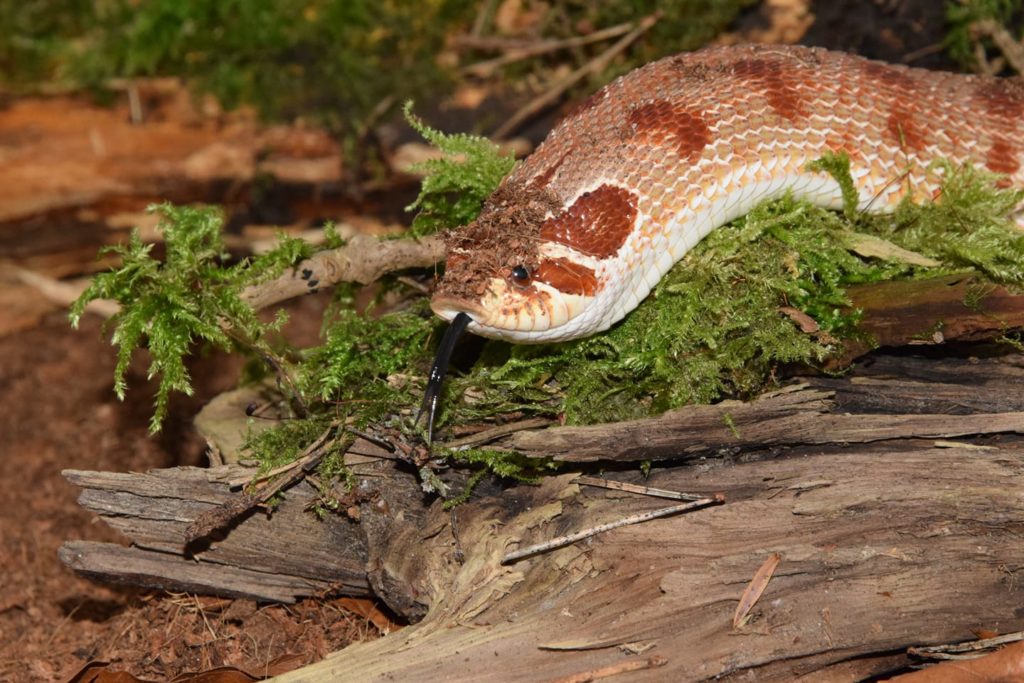This detailed photograph captures a close-up view of a snake's head and upper body, showcasing its texture and distinctive markings. The snake is primarily a brown color with irregular darker cocoa brown patches and dark orange-red spots along its body. Its forked black tongue is prominently extended, adding a sense of motion to the image as it appears to be investigating its surroundings. The snake's head, devoid of any pronounced jowls, suggests it may not be venomous, although caution is advised. The setting is a natural one, with the snake slithering over a richly green moss-covered log, which rests against a backdrop of muted browns and dark ground, possibly littered with some brown debris or dirt. The snake's dark brown eyes are visible, giving it a vigilant expression as it navigates the earthy, forest floor.